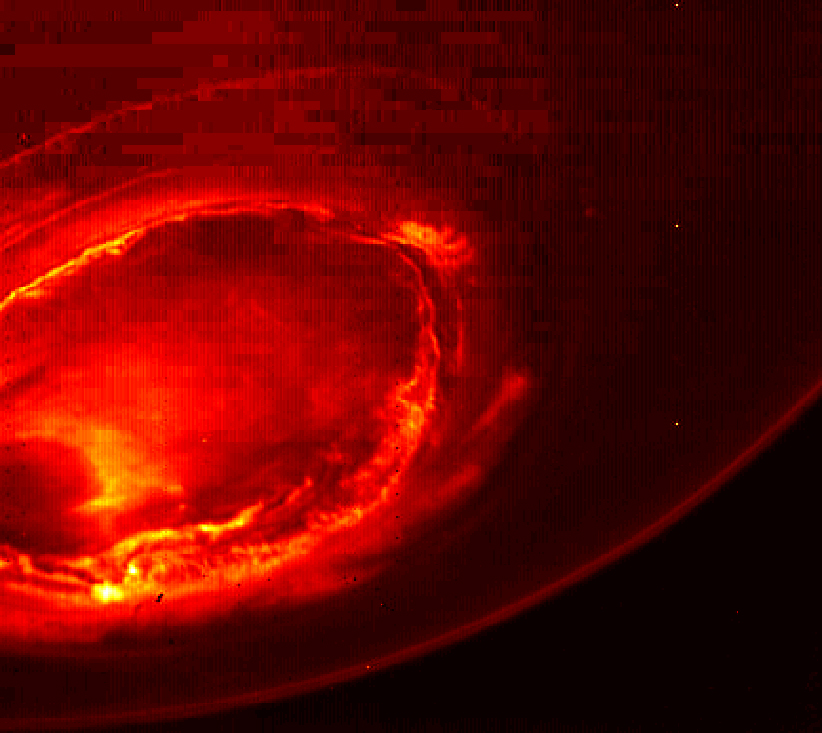The image presents a highly pixelated, square-shaped depiction of a dramatic cosmic event measuring approximately six inches by six inches. Dominating the scene is a large, fiery red orb, which arcs from the lower left, sweeping upwards to the upper left, across to the upper right, and curving back down to the lower left, creating a prominent circular shape. This orb emanates a radiant glow with intense red, orange, and yellow hues, vividly illustrating a high-temperature phenomenon. The center of the orb reveals a concentrated, swirling cloud of yellow and white flames, suggestive of a solar flare or potentially volcanic activity, signifying extreme heat and energy. The backdrop is predominantly black, embellished with a few scattered stars, underscoring the vastness of outer space. The overall effect captures a scene that is both mesmerizing and intensely powerful, radiating a sense of unfathomable heat and dynamic motion.